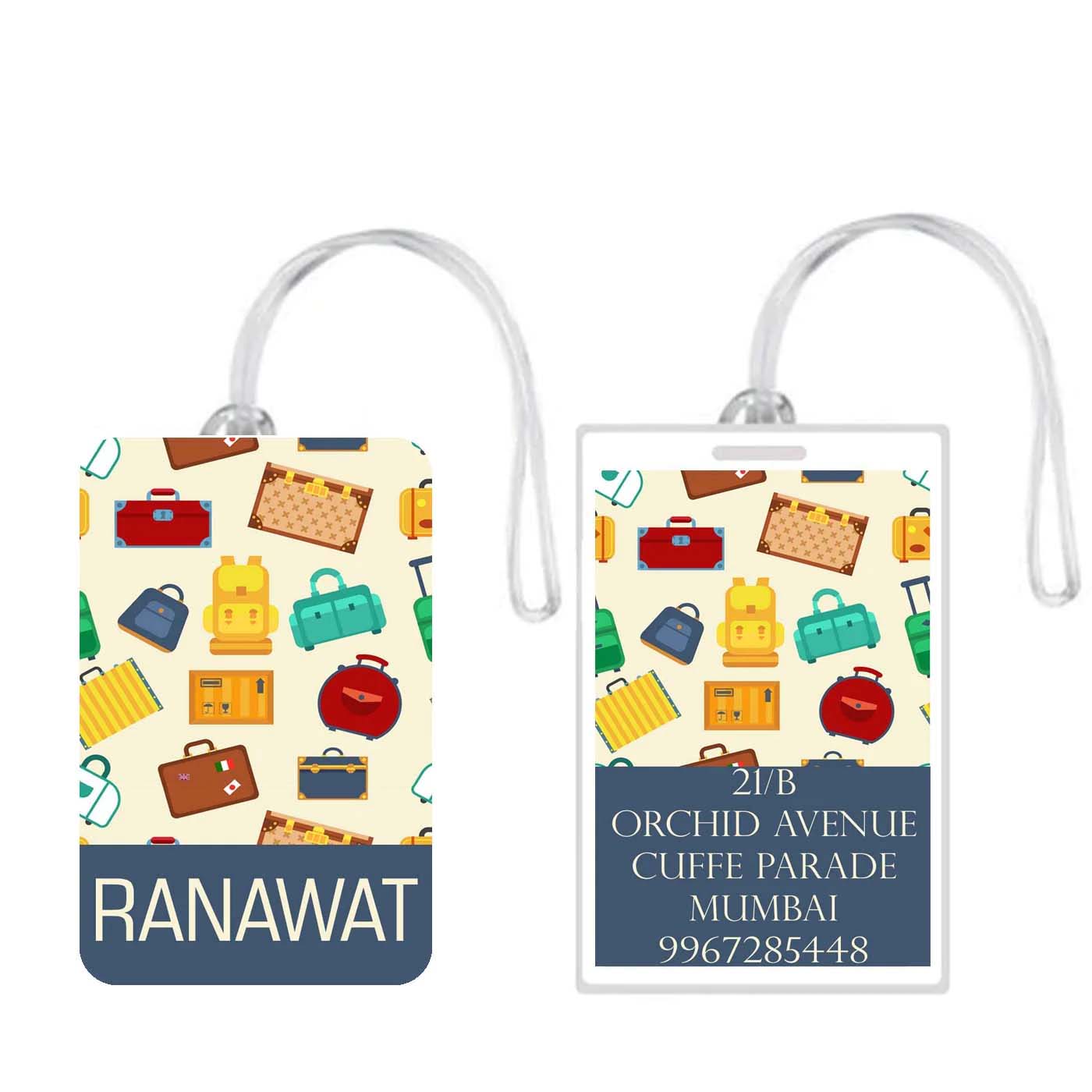The image features two ID tags displayed on a small, clear or white lanyard, set against a plain white background. Both tags showcase a beige background with an array of colorful suitcases, including red, yellow, green, and blue pieces of luggage, along with various handbags. 

The tag on the left is a rectangle with rounded edges and no border, featuring the name "RANAWAT" in large, all-capital white letters on a blue background at the bottom. The tag on the right is slightly more rectangular with a white border and a section on top where a cord could pass through, although the cord does not pass through it in the image. This tag also displays the same luggage pattern on a beige background but is more cropped, with a larger blue rectangle at the bottom containing smaller white text. The text reads: "21/B, Orchard Avenue, Cuff Parade, Mumbai, 9967285448."

Both tags are encased in what appears to be a white or transparent plastic sleeve.